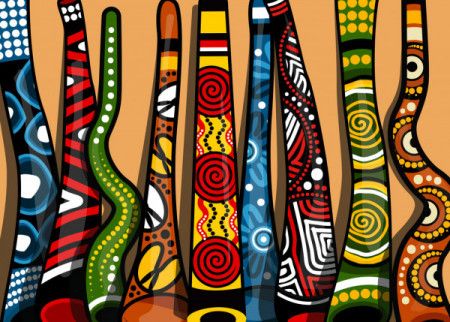The image features a detailed design of nine snake-like shapes set against a tan background, each one resembling a boomerang with unique, vivid designs. These shapes boast a variety of colors and intricate patterns, including stripes, swirls, and geometric shapes. The prominent colors are black, white, blue, red, green, yellow, and orange. One central design stands out with a yellow background adorned with red swirls, interspersed with red, white, and black wavy lines and stripes. Notably, the black boomerang features white polka dots and blue, black, and white circles. Another has distinctive red and white stripes, while yet another has yellow and white dots. There’s a boomerang with red circles connected by black and red lines, a green one adorned with green, white, and yellow circles and lines, and a brown one accented with beads. The detailed artistry of each shape creates a visually dynamic and colorful composition.